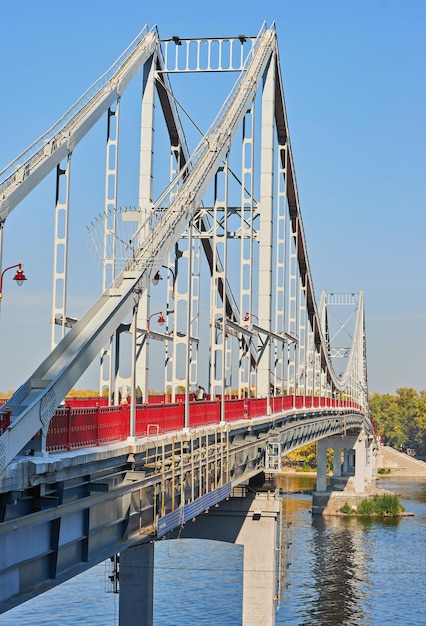This photograph captures a detailed view of a suspension bridge extending diagonally from the bottom left towards the mid-center right, crossing over a body of water. The long, mostly white bridge is supported by concrete pylons extending from man-made islands in the water. It features red barriers on either side to ensure the safety of pedestrians and vehicles. The bridge itself is adorned with red hanging lampposts that illuminate it at night. The perspective of the photo is from the shoreline, providing a side view that reveals the suspension cables connecting to towers along the length of the bridge. Beyond the bridge, an island with a cluster of trees and what appears to be a concrete ramp is visible. The water below has a low and possibly polluted appearance, while the sky above is clear and blue, indicating a daytime setting.